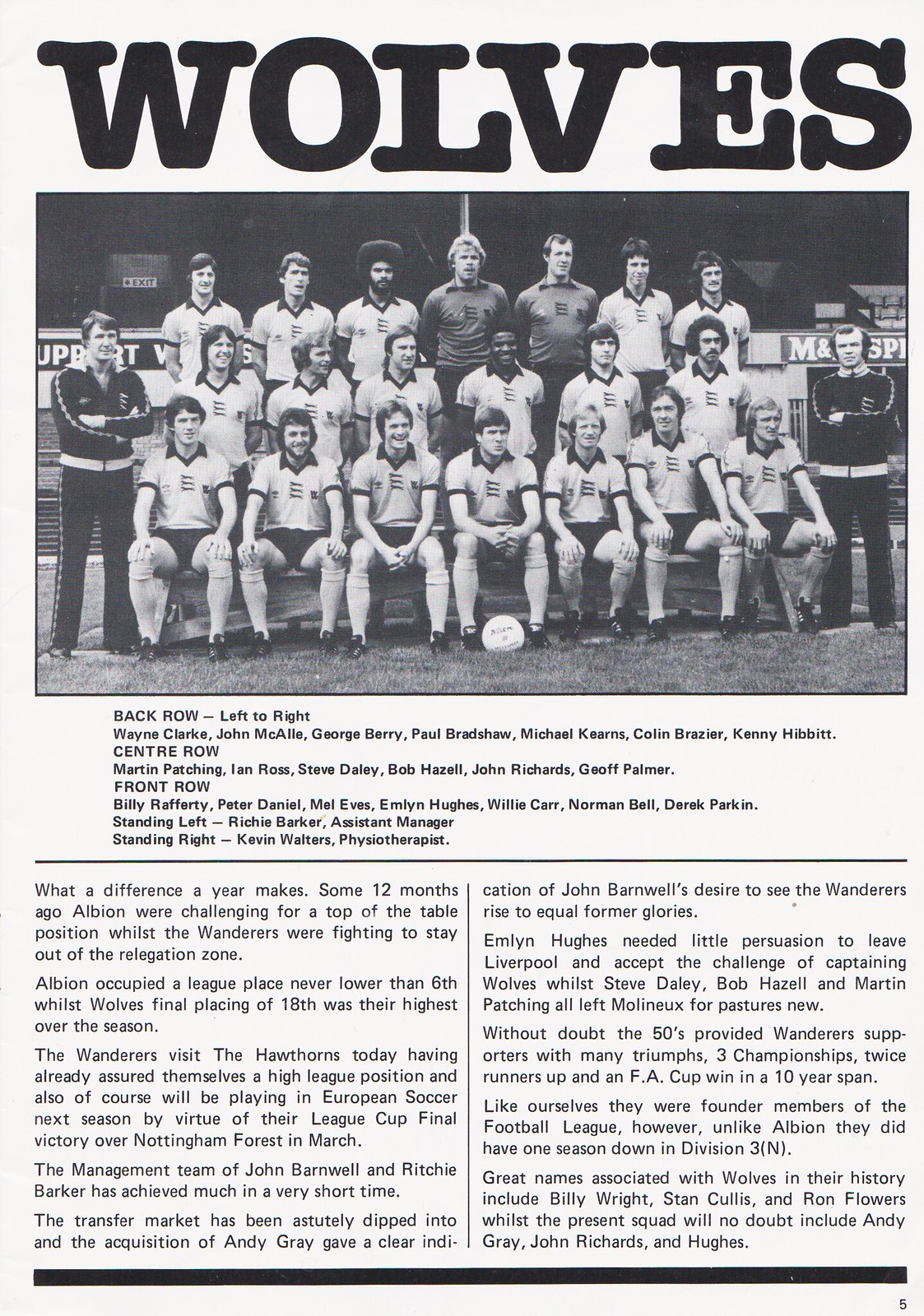This image captures a historical, black-and-white newspaper or magazine article focusing on a soccer team named "Wolves." At the top of the page, the bold, black letters spell out "Wolves" against a white background. Below this headline is a substantial black-and-white photograph of the entire team, consisting of three rows of men. 

In the front row, the players are seated; in the subsequent two rows, the players are standing. The team members are dressed in white shirts with dark collars, dark-colored shorts, and high socks that reach almost to their knees. A soccer ball is placed in front of the seated row. On either side of the photograph, the coaches can be seen standing, adorned in dark-colored track suits. Additionally, two men in gray t-shirts are positioned in the middle of the back row. The team appears to be positioned on the sidelines of a field, with the bottom of the stands visible in the background.

Beneath the photograph, there is a detailed section listing the names of all the team members categorized by their position in the back, center, and front rows. Below this list, two columns of text elaborate on the team's background, performance, and notable events from the past year. The article highlights the turnaround in the Wolves' fortunes under the leadership of John Barnwell and Richie Barker, mentioning their successes, key acquisitions like Andy Gray and Emlyn Hughes, and significant historical achievements. It also contrasts the Wolves' earlier struggles with their more recent successes, including their impending participation in European soccer following a League Cup final victory over Nottingham Forest. The article reflects on the club's storied history, noting famous names and past glories while also acknowledging recent notable players.